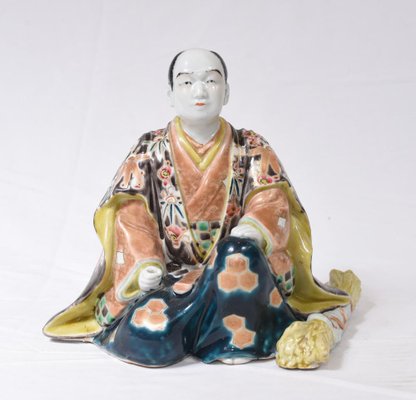This detailed photograph features a Chinese porcelain figurine of a slightly balding man with black hair, sitting on a gray surface against a gray background. The shiny white complexion of the man's face is adorned with red lips and black eyebrows, emphasizing his distinguished Asian features. The figurine is dressed in traditional Japanese-style robes, which are adorned with a multicolored floral pattern, including shades of navy blue, mustard yellow, red, and black. The bottom part of the robe displays red hexagonal decorations. The man appears to be kneeling on his right knee with his left knee slightly elevated, and he holds a small cup in his right hand. To the right of the figurine rests an object resembling a bundle of sticks or a bale of hay. The photograph captures the subtle shadows cast to the side, suggesting the light source is positioned to the left. The intricate details of the floral patterns and traditional attire lend a historic and cultural authenticity to the piece, evoking a sense of religious reverence often associated with Buddha figures.